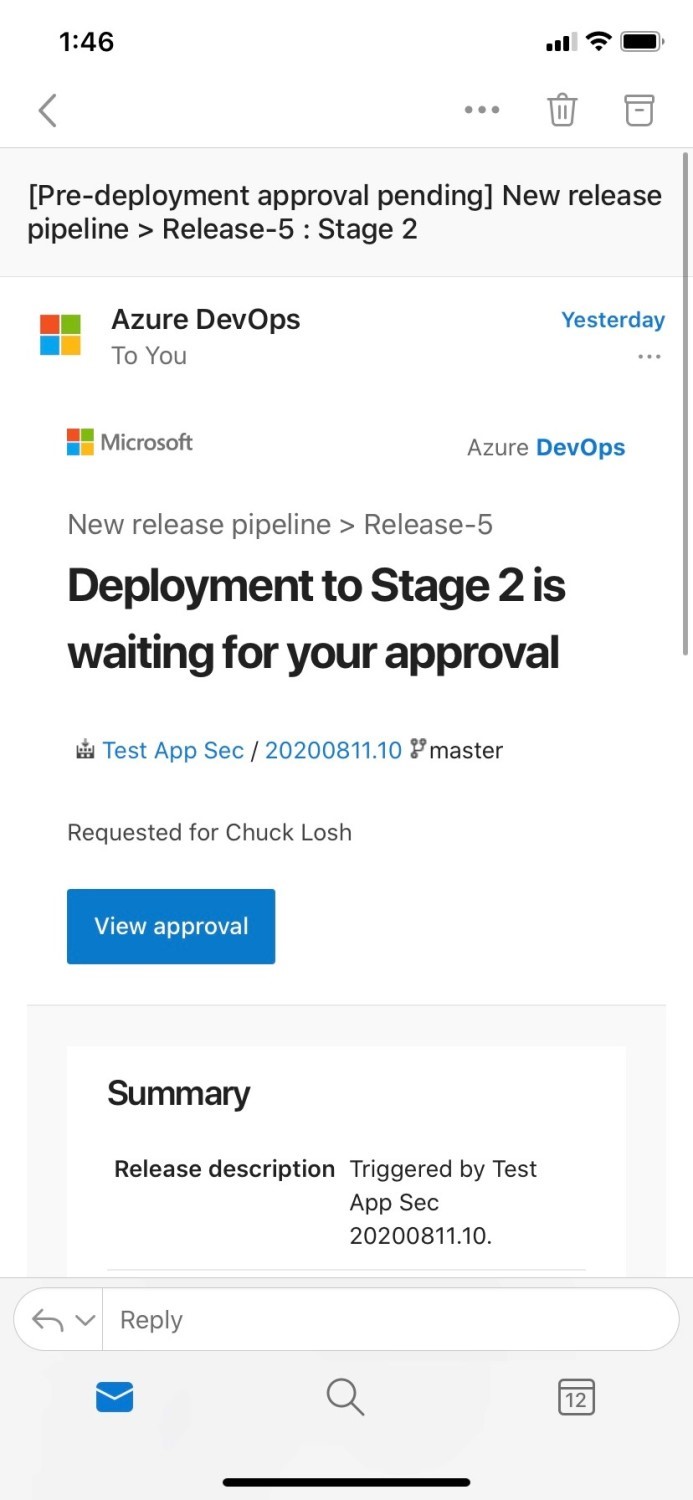### Detailed Caption for the Image:

The image displays a screenshot taken from a mobile device, likely a smartphone, featuring an app interface that appears to be from an email client or a notifications tab related to Microsoft Azure DevOps. 

At the very top of the screen, the device status bar is visible, showing the current time "1:46" on the left side, along with icons indicating battery status, signal strength, and Wi-Fi connectivity on the right side. Just below the status bar, there's a navigation bar including a left-pointing arrow for going back, and three gray icons on the right: a set of three vertical dots, a trash can, and a square icon that might represent a calendar or inbox.

Beneath this navigation bar lies a gray box containing the text: "[Pre-deployment approval pending] Open and close new release pipeline, Release 5, Stage 2."

The main content area is predominantly white, starting with the Microsoft logo on the left and the words "Azure DevOps" next to it, indicating the source of the message. On the right of this line, it states "Yesterday" to indicate the time the notification was sent. 

Below the Azure DevOps title, the phrase "To You" appears, signifying that this message is addressed to the user of the device. Another Microsoft logo followed by "Azure DevOps" further clarifies the sender.

A prominent message in bold black text reads: "Deployment to Stage 2 is waiting for your approval," conveying an urgent call to action. Following this are the details: "Requested for Chuck Walsh." Directly below, there is a blue button labeled "View Approval," offering the user the option to take action.

A summary section is present listing the trigger details, mentioning "Test, App, Second" along with some numerical identifiers. At the bottom of the screen, there is a toolbar housing a search box, a calendar icon, a search icon, and an envelope icon for additional functionalities.

This screenshot appears to encapsulate a critical notification from the Azure DevOps platform, requesting user interaction to approve a deployment step.